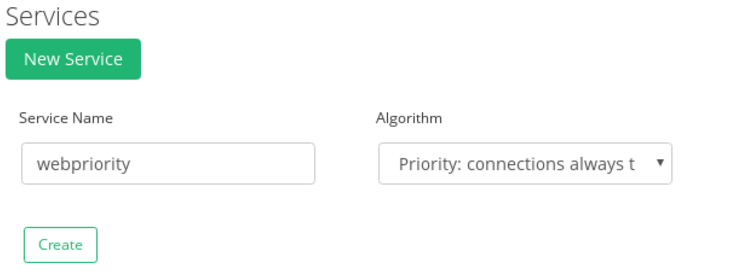This image is a screenshot from a website, focusing on a specific section with minimal context provided. The visible part of the website is set against a white background. 

In the top left corner, the word "services" is written in a gray font. Beneath this, there is a green rectangle with the text "new service" in white font. Below this rectangle, the text "service name" is visible.

Further down, there's a larger rectangle outlined in light gray, containing the text "web priority" written in lowercase letters without any spaces.

On the right side of the page, roughly in the middle, there is a headline that reads "algorithm." Below this headline, there is another rectangular box outlined in gray. Inside, it says "priority: connections always," followed by a truncated word beginning with the letter "T." An inverted black triangle next to this text indicates the presence of a drop-down menu.

Returning to the left side, beneath the "web priority" box, there is a smaller rectangle outlined in green with the green text "create" inside it.